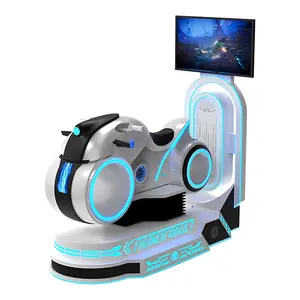The image features a futuristic-looking, white and gray motorbike, adorned with light yellow wheel designs and LEDs, positioned on a mechanical platform that seems to be part of an arcade machine. This setup appears to be part of a motorbike racing game, similar to those found in entertainment venues like Dave and Buster's. The platform is designed to allow players to climb onto the motorbike and interact with the game by riding towards a vertical screen to avoid obstacles. The machine is accented with blue lighting that trims its edges, adding to its modern aesthetic. A monitor is also visible on the top right panel, accompanied by cylindrical components, further enhancing its high-tech appearance.